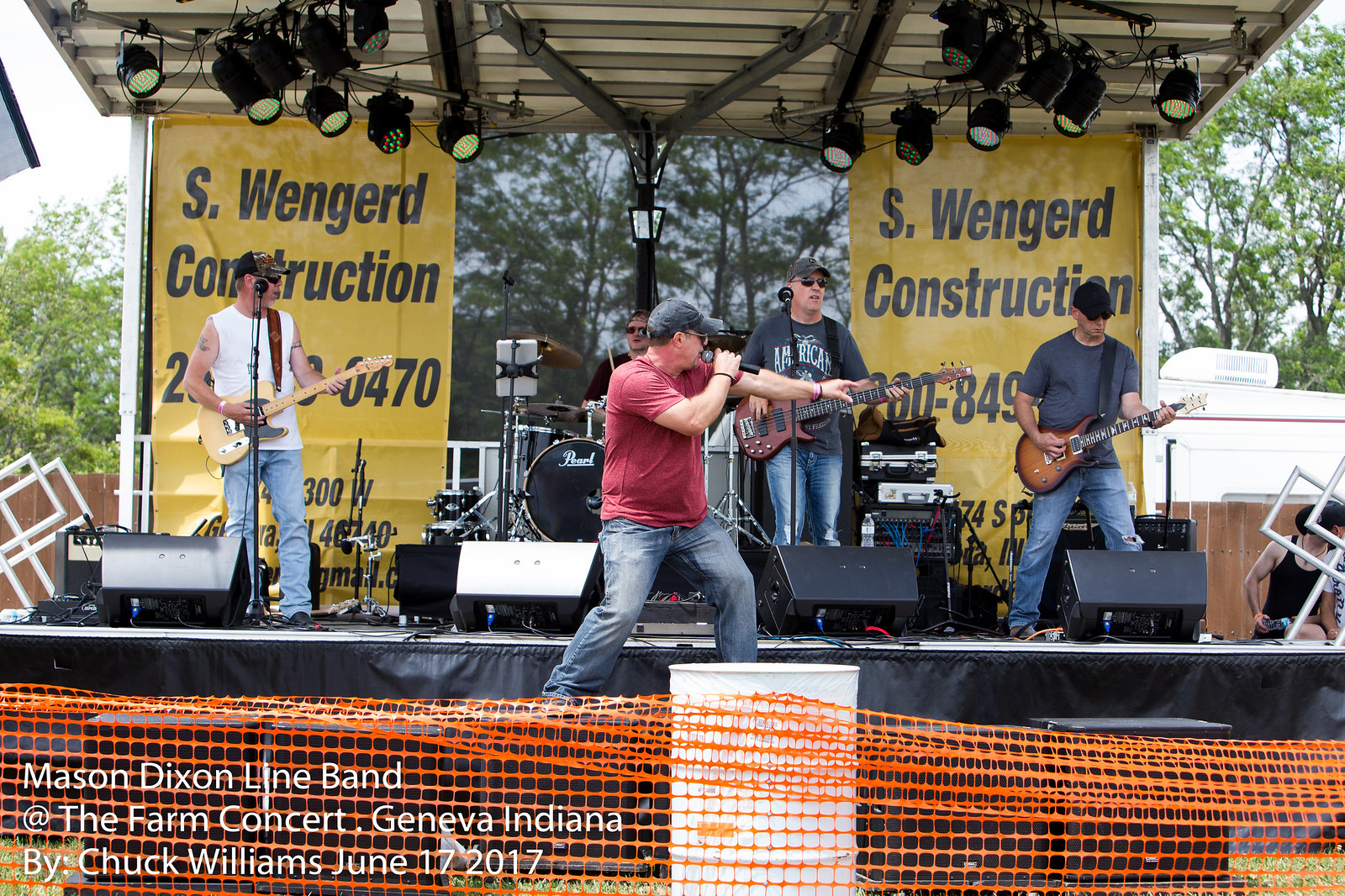This vivid photograph captures an energetic outdoor performance by the Mason Dixon Line Band at the Farm Concert in Geneva, Indiana, taken by Chuck Williams on June 17, 2017. Five men are performing on a small stage, all wearing baseball caps, sunglasses, and blue jeans, fitting the casual outdoor setting under sunny skies. The lead singer, in a red t-shirt and blue jeans, stands prominently at the front, singing into a microphone held in his right hand, while his left arm is extended to the side. He is joined by two guitarists and a bass player, with one guitarist in a white tank top and the others in gray t-shirts. A barely visible drummer completes the lineup behind them. The stage is equipped with speakers, a drum set, and spotlights that enhance the experience, though some appear to be off. In the background, S.Wengerd Construction banners and a phone number are prominently displayed, adding a local touch. The scene is framed by trees, adding to the event’s festive, outdoor ambiance, while an orange plastic fence is visible in the foreground, marking the concert area.